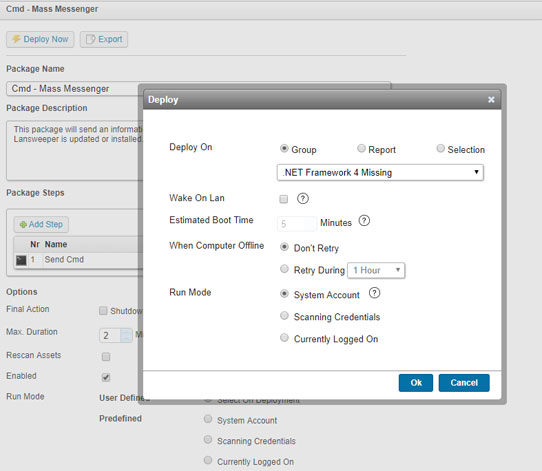The image is a detailed screenshot of a computer application, specifically a control panel for CND-MassMessenger designed for a desktop or laptop computer. The primary focus of the screenshot is on a pop-up window that has emerged, overlaying the slightly grayed-out background interface of the control panel. 

In the upper left corner of the pop-up window, the word "Deploy" is prominently displayed within a gray bar. The body of the pop-up is set against a white background, adorned with black text.

Within the pop-up window, the following details are visible:
- At the top, a section titled "Deploy On" features a selected radio button next to the "Group" option.
- Adjacent to this, two buttons labeled "Report" and "Selection" are positioned to the right.
- Below this setting, a drop-down menu shows ".NET Framework 4 Missing" as the selected option.
- A list of options runs down the left-hand side of the pop-up:
  - "Wake On LAN"
  - "Estimated Boot Time: 5 minutes"
  - For the "When Computer is offline" setting, the radio button for "Don't Retry" is selected.
  - "Run Mode," with "System Account" chosen as the option.

Finally, in the bottom right corner of the pop-up, two prominent blue buttons are visible, labeled "OK" and "Cancel."